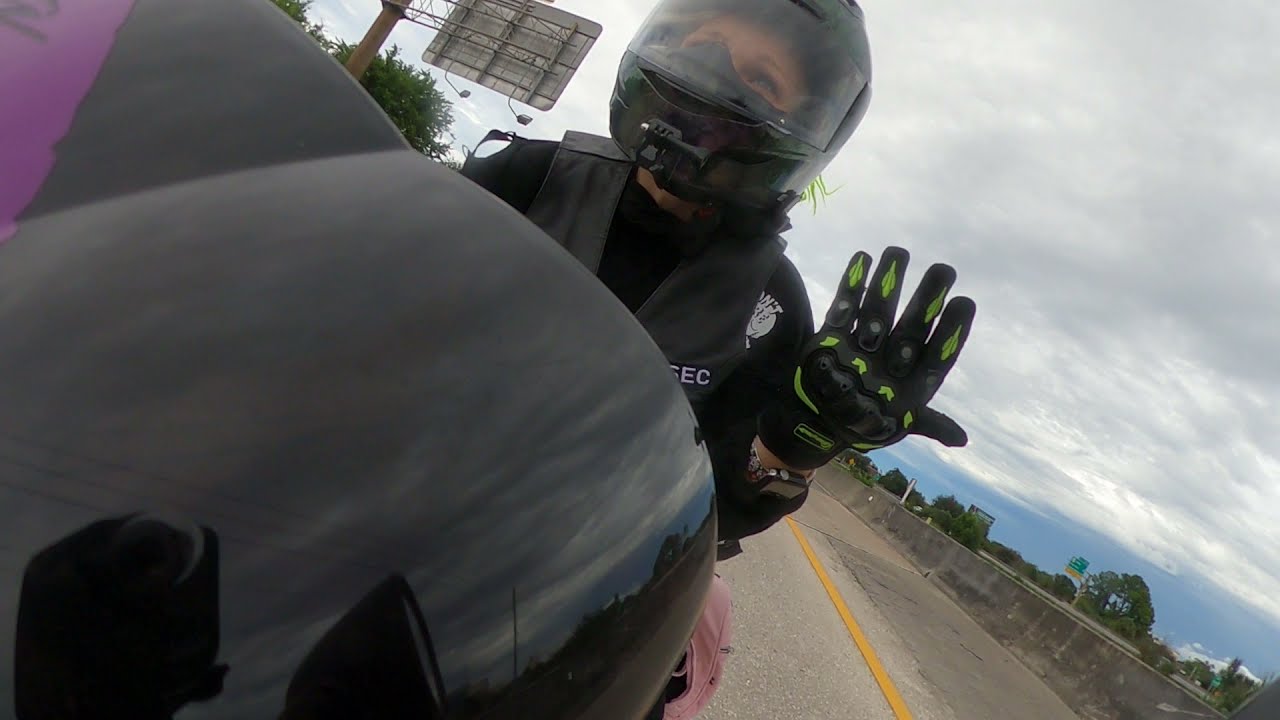In this close-up image, a female motorcyclist is prominently positioned at the center of a black motorcycle, with the front of the bike visible on the left-hand side. She dons a black helmet with hair peeking out the back, and her face is partially visible, showcasing her eyebrows and makeup. Her attire includes a black shirt, a black vest with "S.E.C." written in white on the right-hand side, and black gloves featuring green accents. Remarkably, she is holding up her right hand, with fingers and thumb extended, possibly for a gesture. A harness or backpack is visible on her back.

The setting is a freeway, evidenced by the highway sign on the left and the yellow-striped road to the right. Additionally, there is a concrete barricade wall to the right, behind which are trees. The sky above is filled with white and grayish clouds. The photograph appears to be taken from a mounted perspective, possibly a GoPro attached to the motorcycle, giving a wide-angle view of the scene.